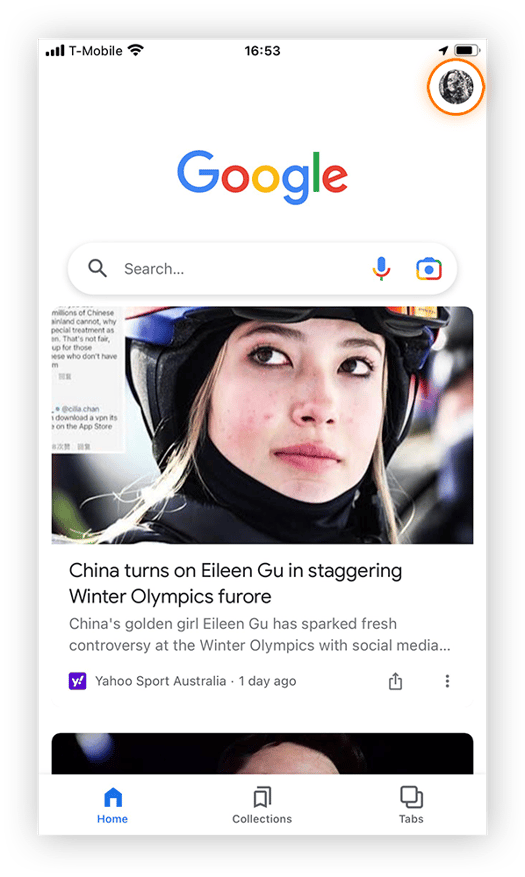This image is a detailed screenshot taken from a smartphone in portrait mode. In the upper left corner, the network provider is indicated as T-Mobile. The upper center displays the time as 16:53, while the upper right-hand corner shows a battery icon that is more than 50% filled next to an avatar. The avatar, which is enclosed in a white circle, has an additional hand-drawn orange circle around it, drawing attention to this specific element on the screen.

Below this, the interface displays the Google logo followed by a search bar. Featured prominently is a large image of a woman, possibly a race car driver, with light skin and facing towards the left side of the image. The accompanying text reads, "China turns on Aileen Gu in staggering winter olympics furor." Further details reveal: "China's golden girl Aileen Gu has sparked fresh controversy at the winter Olympics with social media," sourced from Yahoo Sports Australia, one day ago.

Further down, there is a glimpse of another image with a blue background and what appears to be either a bald head or dark hair. The bottom left corner of the screen indicates that the user is on the homepage, as denoted by the illuminated blue home icon. There are also two other sections labeled "Collections" and "Tabs," which users can navigate to.

Of particular interest in the image is the hand-drawn orange circle around the white-encircled avatar in the upper right-hand corner. Despite other details on the screen, the standout feature is the highlighted news headline about Aileen Gu, marking it as the primary news topic of the day, possibly focusing on sports news.